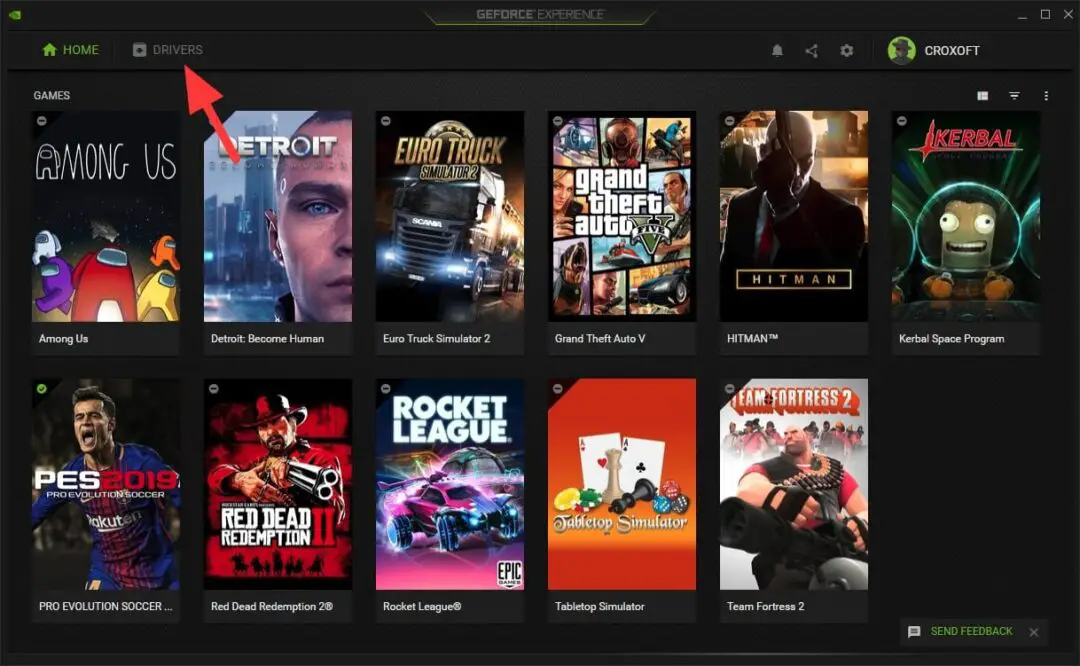The image captures a screenshot of a computer monitor displaying a software interface, specifically the GeForce Experience dashboard. At the top, the interface features a header with a green 'Home' button, alongside tabs for 'Drivers' and 'Games.' 

Within the 'Games' section, there are two rows of game titles. The top row consists of six games, starting with "Among Us," followed by "Detroit," "Euro Truck Simulator," "Grand Theft Auto," "Hitman," and "Iceball." The bottom row contains five games: "PES 2019," "Red Dead Redemption 2," "Rocket League," "Tabletop Simulator," and "Team Fortress 2." There is an empty space in the lower-right corner of the grid, indicating a missing or unlisted game.